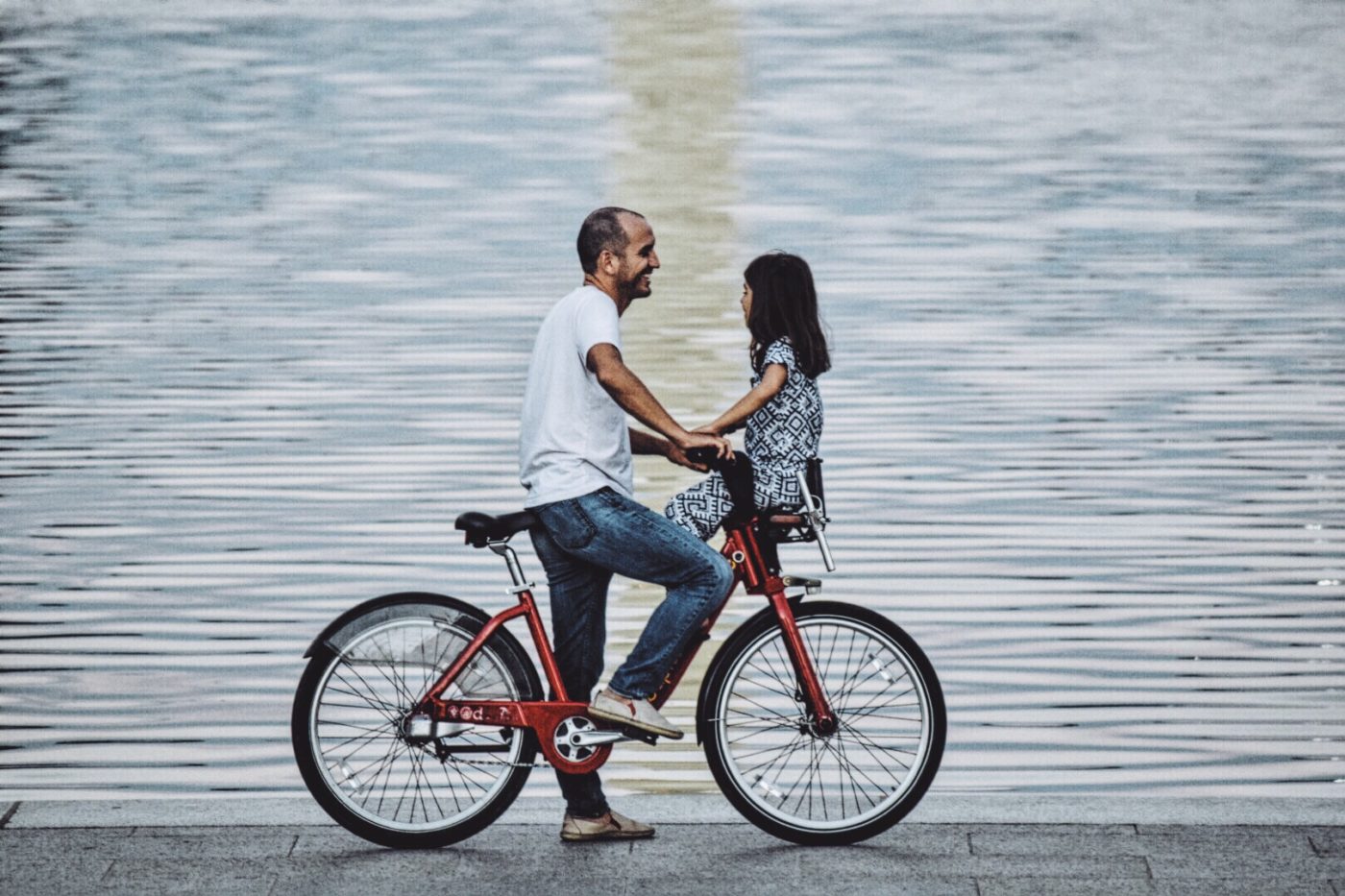The image depicts a touching scene of a man and a young girl on a red bicycle, positioned on a concrete pathway beside a body of water, likely near a famous monument featuring a reflecting pool and a tall white tower in the distance. The man, dressed in a white t-shirt, blue jeans, and white and red tennis shoes, is standing with his left foot on the ground and his right foot on the pedal, hands on the handlebars. Directly in front of him, the young girl, possibly five or six years old, sits in a specialized front attachment that faces backward so she can easily converse with him. Her outfit consists of a blue and white, or black and white, patterned dress or blouse and shorts, and she has brown hair. They are smiling warmly at each other, sharing a moment of joy. In the background, the rippling water and the stone path create a serene setting for this heartwarming interaction.